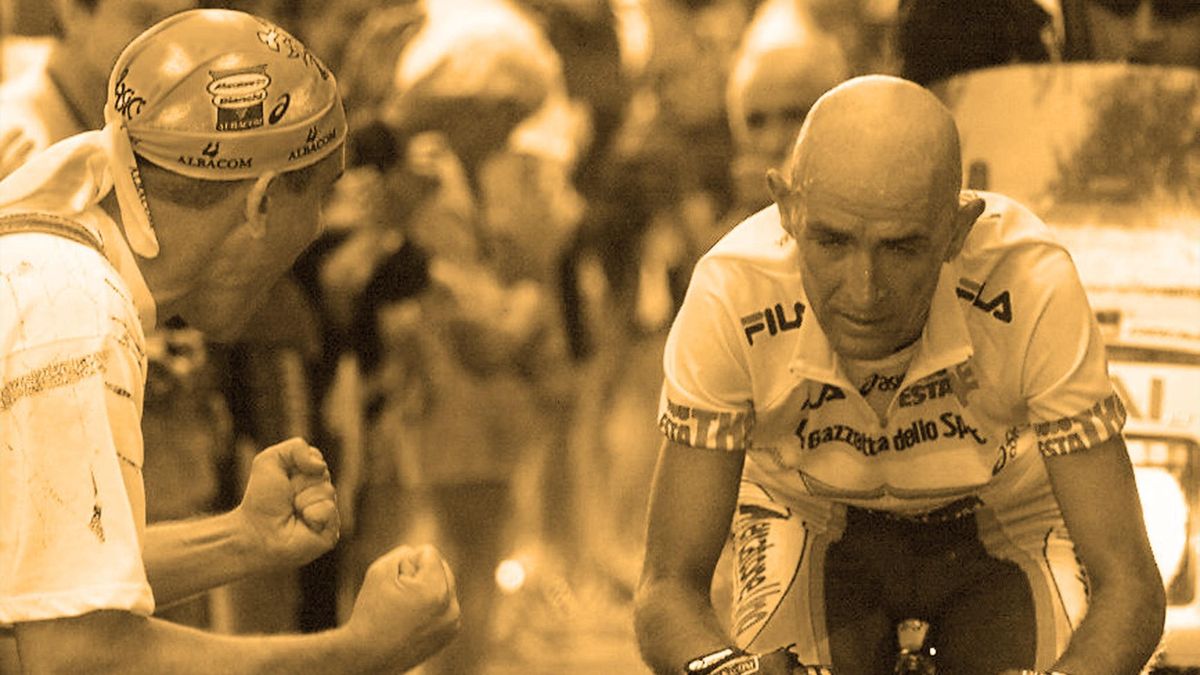In this black-and-white photograph, the focal point is a determined, bald man, sweaty and slightly hunched over, riding a bicycle towards the camera. He is dressed in cycling gear: a white, short-sleeved Fila t-shirt, visibly soaked and wrinkled, with a zipper down the front and black and gray lettering on the sleeves, and black, white, and gray biker shorts adorned with indistinct writing. To his left, a man in his 40s or 50s, wearing a white t-shirt and a distinctive bandana emblazoned with "ALBACOM," is enthusiastically cheering him on, his fists clenched tightly in a gesture of encouragement. In the background, partially visible, is a man on a white motorcycle with a glass shield, wearing sunglasses. The scene is vivid despite being in monochrome, capturing the raw intensity and support within the competitive race. Blurred figures cheer along the route, adding depth and energy to this compelling moment.